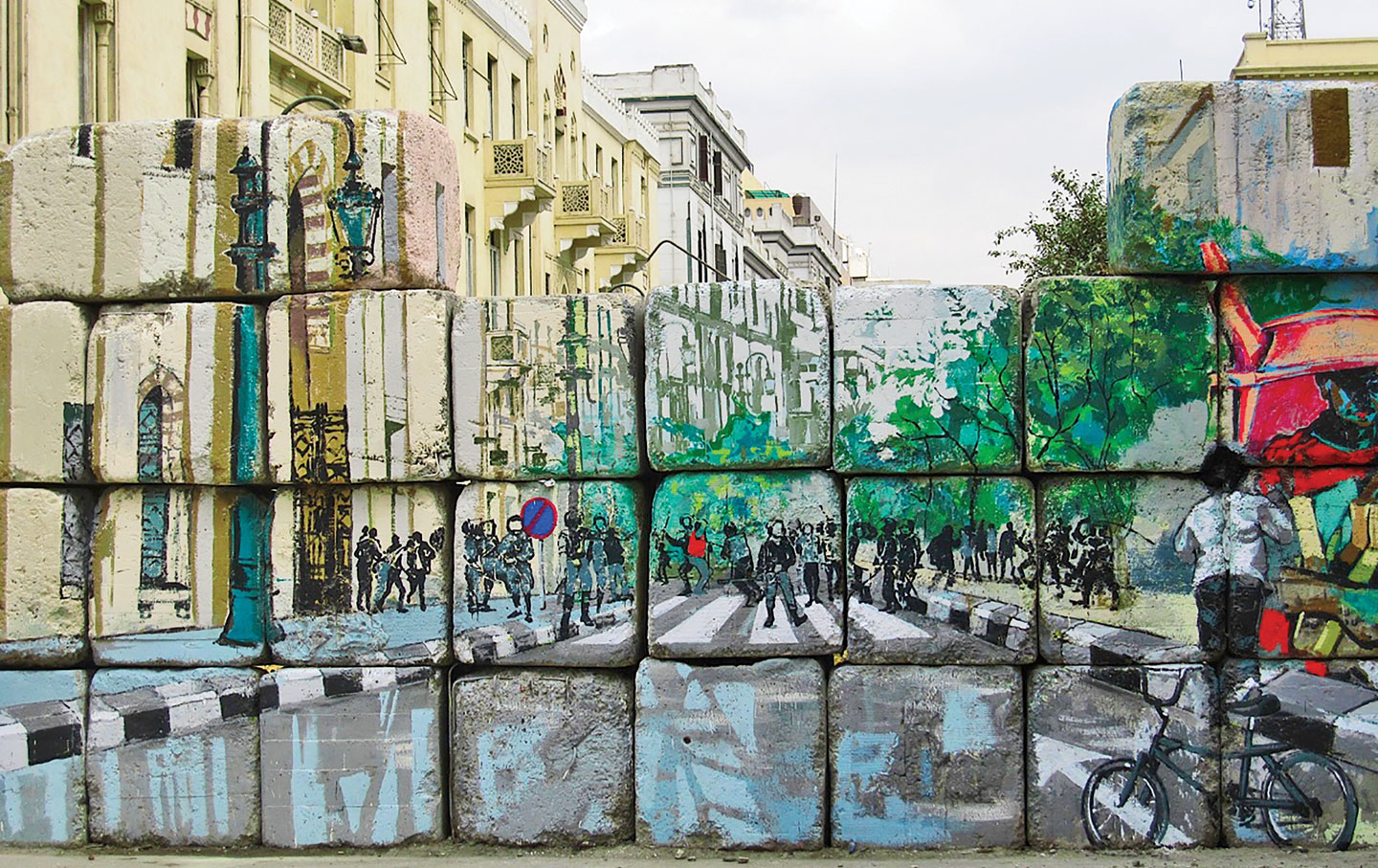In this rectangular, wide photograph, the foreground features several layers of square ceramic bricks that have been intricately painted to form a mural. This mural cleverly depicts an extension of the street behind these blocks, creating an illusion of a continuous scene. Each brick has been painted to align seamlessly with the background, which showcases a row of mid-rise buildings, predominantly yellow and gray, under a gray, overcast sky. The mural itself depicts a vibrant street scene with people, possibly police or military personnel, some with riot batons, standing amidst the crowd. On the right side of the image, a person is seen standing near a bicycle next to a colorful object with a spout. The overall effect is a striking blend of art and reality, making the painted blocks appear as transparent windows into the actual street behind them.